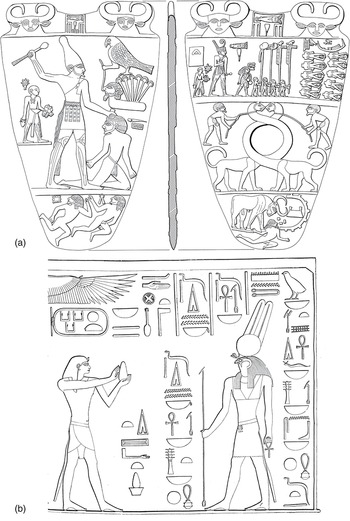This highly detailed black and white illustration represents ancient Egyptian art and hieroglyphics, divided into two main sections labeled A and B. 

The top section (A) displays two separate but thematically related vignettes resembling the shapes of shields or vases, each filled with intricate imagery. 

On the left, the depiction features a shirtless pharaoh holding a stick in one hand and seemingly about to strike a man kneeling before him, possibly a slave. This imposing figure is adorned with traditional attire and a headpiece, and a falcon perches above him. In the background, smaller figures can be seen, emphasizing the pharaoh's dominance. Below this scene, two more people are depicted, possibly involved in an act of worship or servitude.

On the right, the second vignette is similarly detailed but contains different imagery. A line of small and tall figures, potentially representing a procession, stands prominently. Beneath them, two fantastical creatures with intertwining long necks appear, adding mythological elements to the scene. At the base, a bull and a human figure are shown, suggesting themes of domestication or sacrifice.

The bottom section (B) features a squared-off frame filled with hieroglyphics and two facing figures. The figure on the left is drawn in traditional Egyptian style, with raised arms holding unspecified objects. The hieroglyphs are meticulously arranged above and between the characters, as well as down the right side of the square. Across from the first figure, a second, possibly deity-like figure, stands facing left, gripping a long, thin rod and an ankh. 

Throughout the illustration, the artwork maintains a light gray tone, lending it a delicate, ancient parchment-like quality. The precise lines and detailed forms suggest the craftsmanship of ancient Egyptian artisans and provide a glimpse into their complex societal and religious structures.